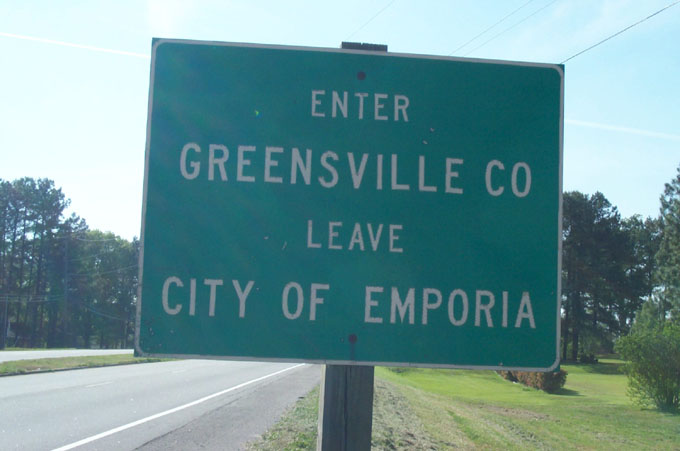This detailed photograph captures a well-maintained, four-lane divided highway with clearly visible white shoulder stripes and an exceptionally manicured grassy median. The scene is set on a bright, sunny day with a vibrant blue sky. Lines of trees—predominantly pine and some deciduous—adorn both sides of the road, providing a lush, green backdrop. The focal point of the image is a standard green and white city limit sign positioned along the grassy shoulder. This sign, mounted on a wooden post, reads "Enter Greensville Co. Leave City of Emporia," clearly marking the border between the two municipalities. The grass along the median and shoulder is meticulously mowed, giving the area a tidy, almost pristine appearance, reminiscent of a well-kept golf course. The absence of buildings and traffic emphasizes the tranquility and natural beauty of the setting.